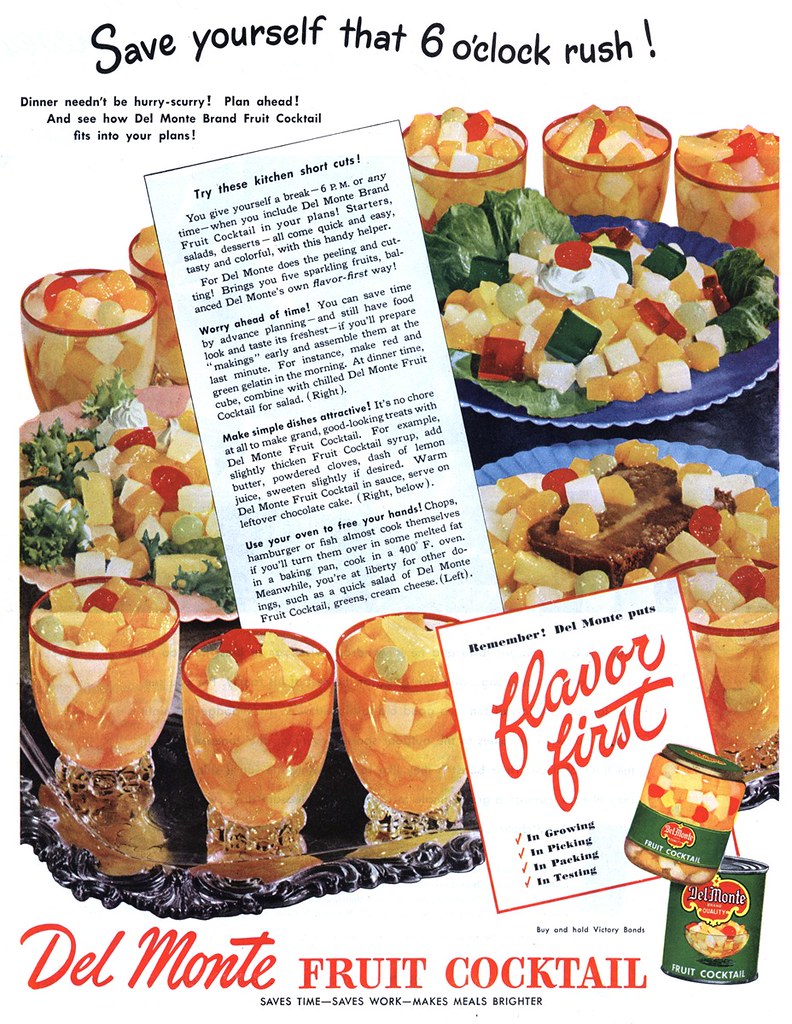This detailed and vibrant magazine advertisement from the 1960s for Del Monte Fruit Cocktail is designed to catch the eye with its colorful photographic elements and persuasive text. At the top, in bold black font, the ad declares, "Save yourself that six o'clock rush!" and follows with smaller text instructions, "Dinner needn't be hurry scurry. Plan ahead and see how Del Monte brand fruit cocktail fits into your plans."

The central image displays a sumptuous arrangement of small, clear, footed dessert glasses, each rimmed with gold or red and filled with Del Monte's vibrant canned fruit cocktail, featuring cherries, grapes, peaches, and pineapples. These glasses are artistically arranged on a rectangular, silver-plated tray with ornate edges. About five glasses are clearly visible at the front, with more suggested behind a superimposed text block that covers part of the back.

Nestled in the middle of the tray are three scallop-edged blue plates, one with large lettuce leaves topped with a whimsical dessert of jello chunks, fruit salad, whipped topping, and a maraschino cherry. Another plate hosts a composed salad featuring chunks of fruit salad around what appears to be a piece of meatloaf or pork chop. The third plate holds yet another artistic fruit salad arrangement.

In the bottom right corner of the image, two small cans of Del Monte Fruit Cocktail are displayed next to a bold message in red and black: "Remember! Del Monte puts flavor first." This motto is further emphasized by a tagline in large red letters, "Save Time - Save Work - Makes Meals Brighter," promoting the practical advantages of using Del Monte products. Across the bottom of the ad, a newspaper-like text block offers various kitchen shortcuts, reaffirming how Del Monte Fruit Cocktail can simplify meal preparation while enhancing the dining experience.